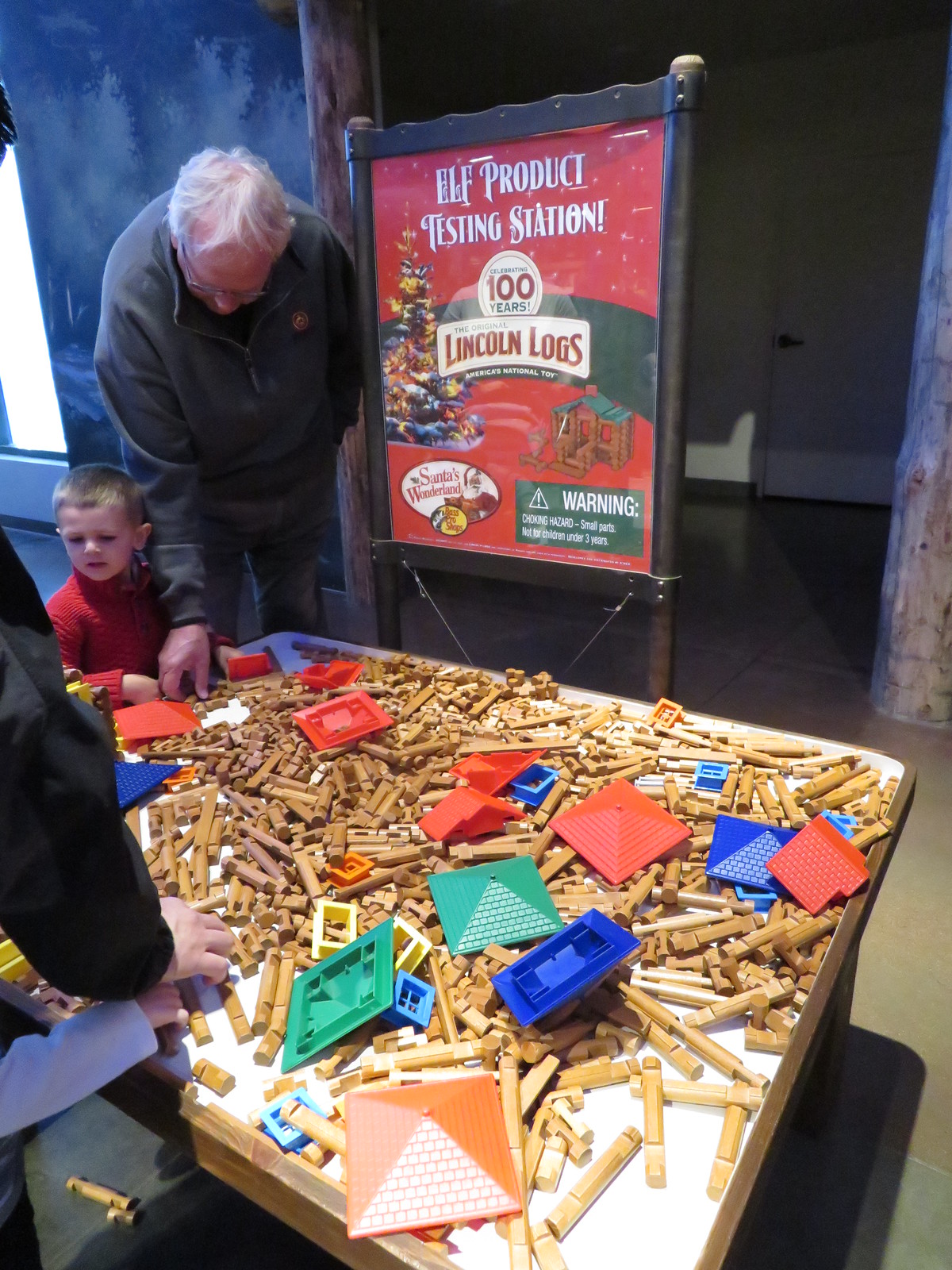In this festive scene, a white table with raised edges is filled with an assortment of tan, brownish, rounded wooden pieces, reminiscent of Lincoln Logs. The table surface is designed to look like tiled roofing in red, green, and blue, adding a playful, log cabin aesthetic. In the background, a bright red poster adorned with a colorful Christmas tree to the left declares "Elf Product Testing Station - 100 Years of Lincoln Logs" in bold white letters. An older man, clad in a gray sweatshirt, bends over the table, touching one of the wooden logs, while beside him, a young boy with blonde hair, wearing a red sweatshirt, watches intently. This image captures a moment of intergenerational connection and creativity during the holiday season.